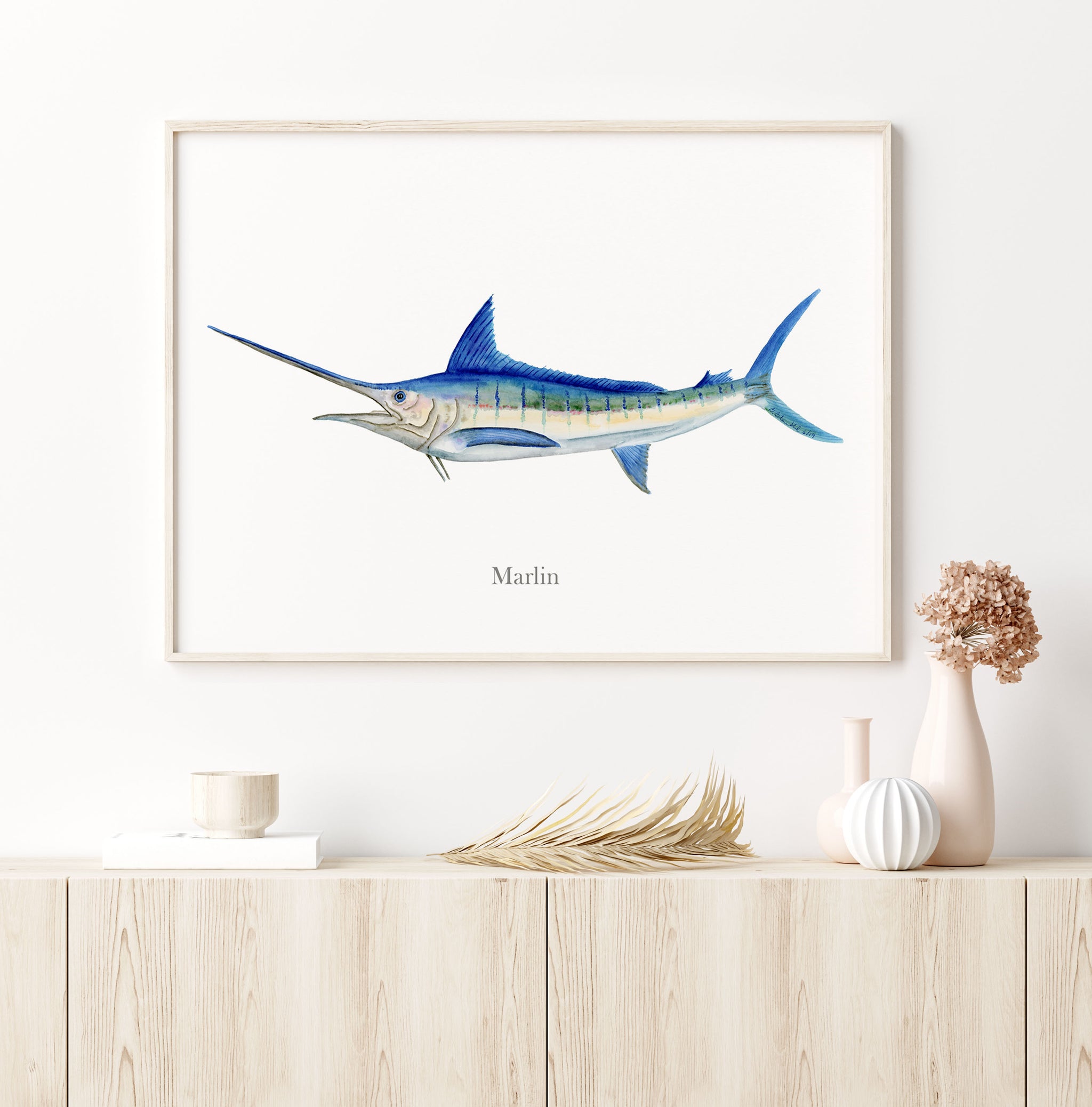The image features a painting of a marlin hanging on a white wall. The marlin, depicted with a sharply pointed nose and a pointed lower jaw, boasts brilliant blue dorsal and tail fins. The top half of the fish is predominantly blue, while the lower half transitions into beige and a light grayish-blue shade. A green stripe runs along its side, adding to its vibrant coloration. The word "marlin" is inscribed below the fish within the painting. Directly beneath the artwork, an off-white wooden table with brown wood grain details holds a white vase filled with flowers, a circular white object, a cup or mug, and a light yellow grass-like decor. The scene captures the elegance and detail of both the marlin painting and the tastefully arranged items on the table below.